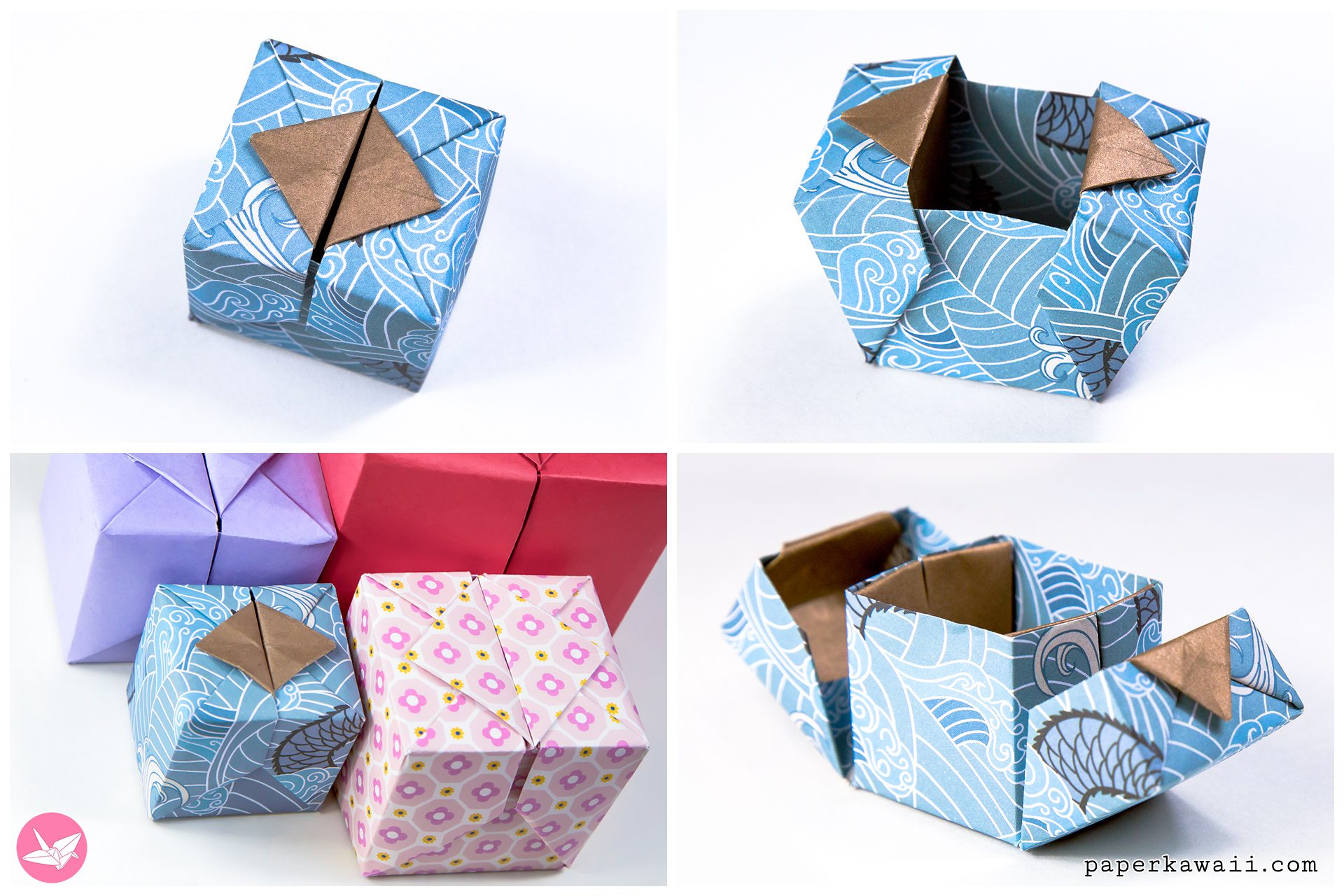The image is divided into four sections, showcasing various gift boxes designed by PaperKawaii.com. In the upper left panel, there is a closed box crafted from blue and white paper with a brown diamond on the top. The panel to the right displays the same box opened, revealing its intricate fold-out design. The bottom left section shows four different closed gift boxes: one in the original blue and white design, another in solid lilac, a third in solid reddish, and the fourth in a multicolor pattern of white, lilac, and yellow. The bottom right panel illustrates the blue and white box opened even further, expanding like a flower to reveal its cardboard interior lined with wrapping paper. The designs emphasize artistic origami elements, meant to promote the creator's unique gift wrapping solutions. All sections prominently feature the PaperKawaii.com watermark.